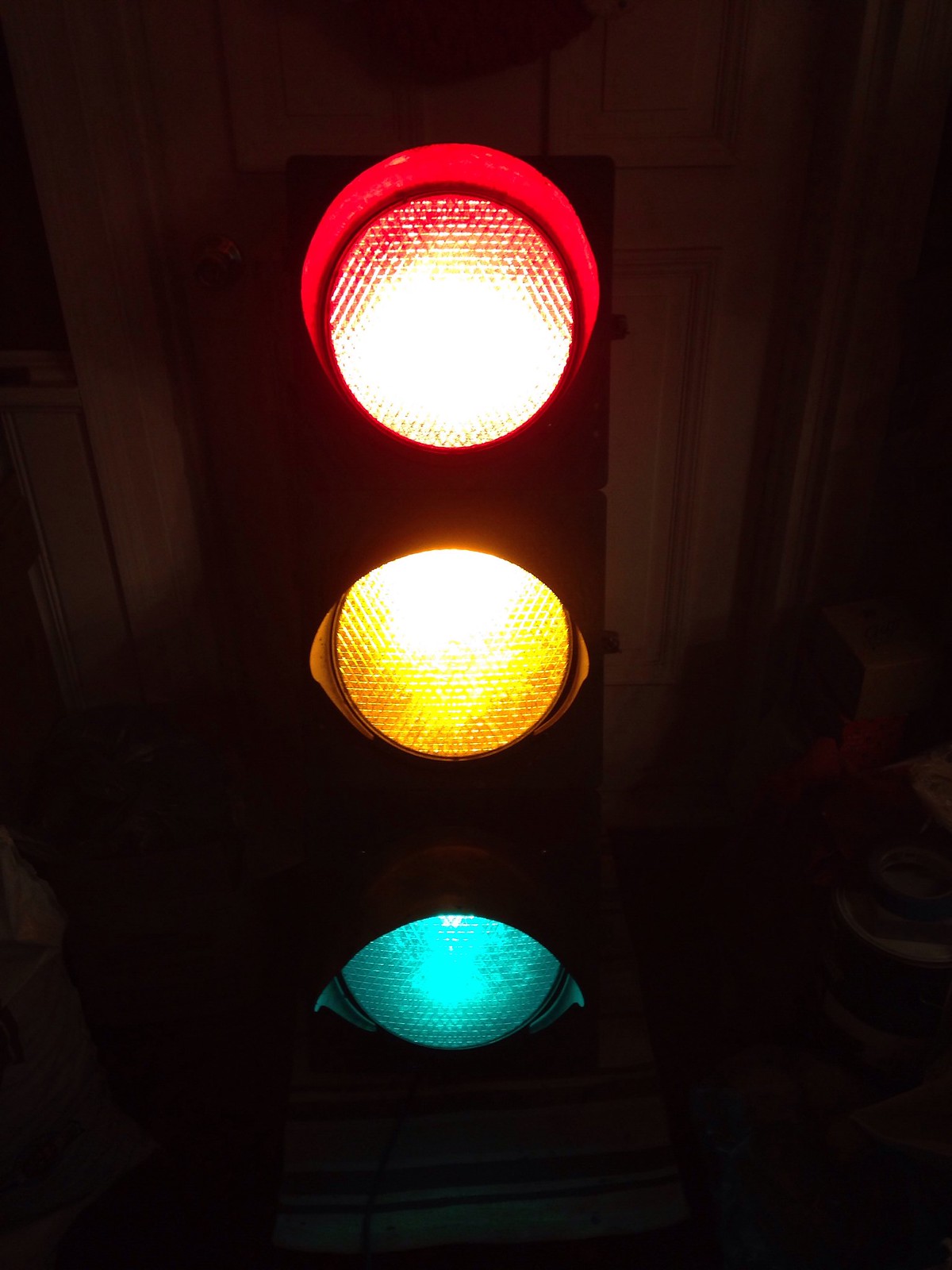This detailed photograph captures a traffic light prominently against a pitch-black background, creating a stark contrast that emphasizes the light emitted from the traffic light itself. All three lights—red at the top, yellow in the middle, and green at the bottom—are illuminated simultaneously, casting a muted glow in their respective colors. The red light, which is the largest due to the slight downward angle of the shot, features a checkered glass lens and appears fully circular, whereas the yellow and green lights are more oval or eye-shaped. The lenses of all three lights share a checkered pattern and each light has a top cover that directs the illumination downward.

The setting appears to be indoors, hinted at by the presence of indistinct wooden structures and a barely visible white door behind the traffic light. This artistic photograph was likely taken inside a room, with the traffic light positioned against a wooden backdrop or possibly mounted to a stand, though this is not entirely clear due to the darkness enveloping the background. The overall ambiance is heavily shadowed, with the traffic lights themselves being the primary source of illumination, casting enough light to reveal some vague details in their surroundings. The green light has a slightly bluish tint, adding to the unique atmosphere of the image.